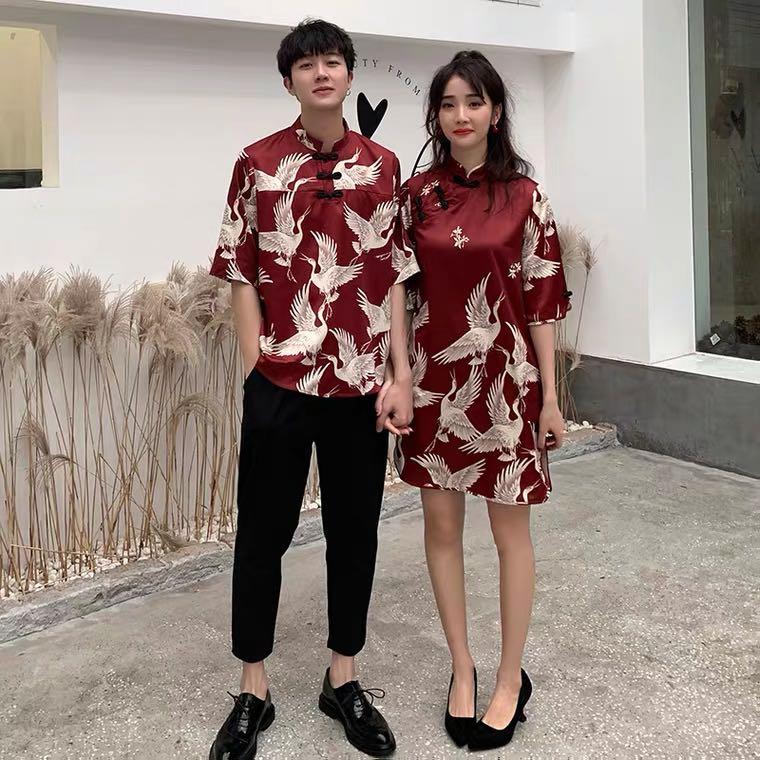This color photograph captures an Asian couple posed together on a concrete path, holding hands. The young man stands on the left, smiling and wearing a maroon shirt adorned with a pattern of white cranes, featuring a Mandarin collar. His short black hair contrasts with his black ankle-length pants and shiny black lace-up dress shoes, worn without socks. His left hand is tucked into his pocket. The young woman stands on his right, appearing slightly uncomfortable. She has black hair styled in a half ponytail reaching her shoulders, accentuated by her red lipstick. Her burgundy dress mirrors the crane pattern of the man's shirt and also features a Mandarin collar, ending above her knees. She complements her outfit with black high-heeled shoes featuring pointed toes. Behind them stands a white wall with a black heart between their heads, and dried tall grasses with feathery ends can be seen to the left.